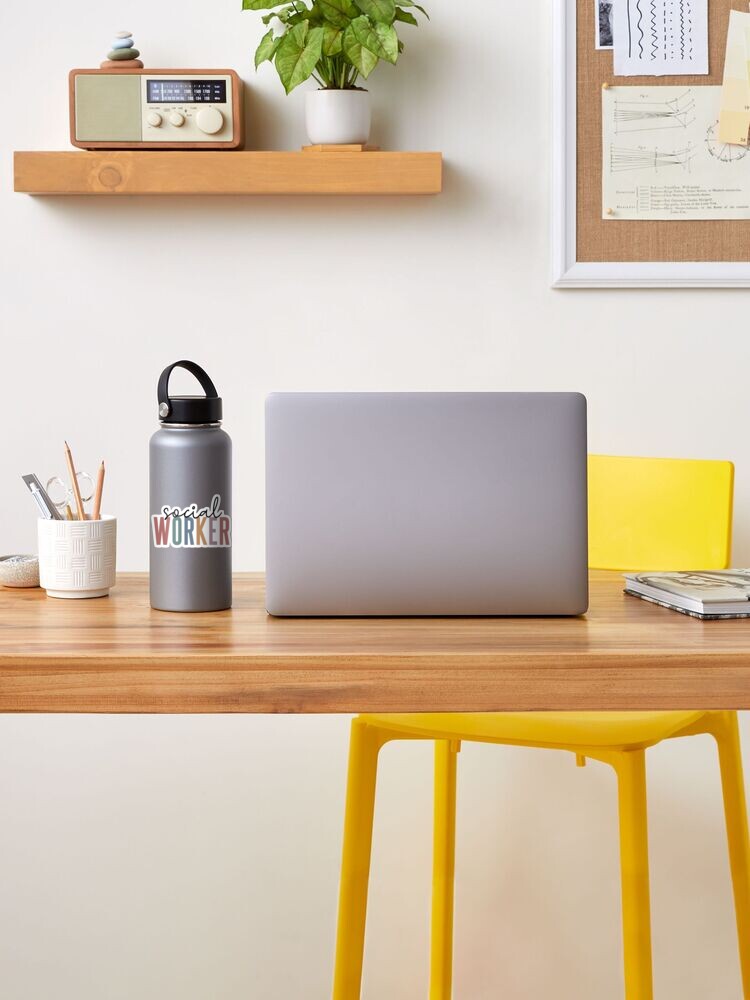The photograph, reminiscent of a staged catalog scene, captures a neatly arranged workspace bathed in natural daylight. The focal point is a light brown wooden desk, perhaps made of pine, paired with a distinctive tall yellow four-legged chair featuring a shorter back. On the desk, an open, plain silver laptop is accompanied by a matching silver thermos adorned with a "social worker" sticker and a black lid. To the left of the laptop, a white ceramic mug serves as a pen holder, containing scissors, a utility knife, and some pencils. A notebook lies on the right-hand side of the desk.

The white wall behind the desk is adorned with a white-framed corkboard hosting several pieces of paper with drawings and notes pinned onto it. Above this, a wooden shelf holds an array of items: an old-fashioned dial radio with a pile of river stones on top, a small potted plant in a white planter, and a retro alarm clock. The thoughtful arrangement and cohesive color palette of the workspace elements create an inviting and efficient atmosphere.